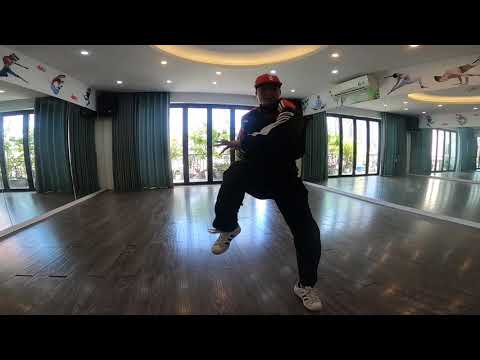The image depicts an indoor dance studio featuring a single male dancer mid-jump, likely performing a hip-hop routine. He is dressed in a black sweatshirt, black pants, a red baseball cap, and white tennis shoes. The dance studio is well-lit, with brownish-grayish flooring. Both the right and left walls are completely covered with large mirrors, reflecting the dancer's movements. In the background, there are floor-to-ceiling windows covered by open curtains, slightly blurry, revealing a distant view of trees outside. The clarity of the image is mostly sharp, though some parts appear distorted and blurry, especially the background. The setting emphasizes the dynamic energy and space of the dance studio.